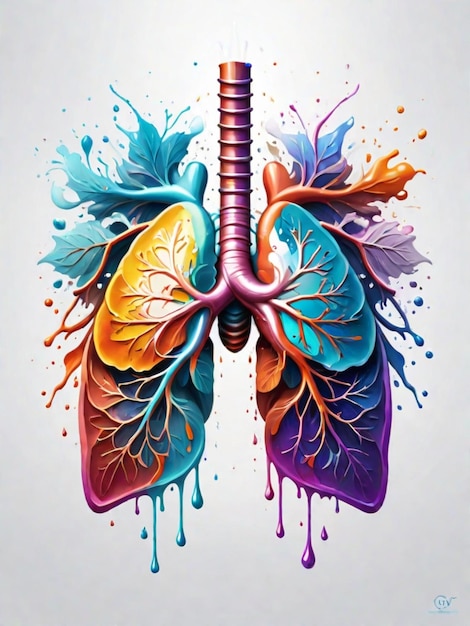This is a detailed and vibrant painting of the human respiratory system, focusing on the lungs and windpipe. The trachea, depicted as a brownish tube with a whitish glow, descends and splits into the bronchial tubes, leading into the left and right lungs. The lungs are portrayed with unique color schemes: the left lung features a blue top and a purple bottom, whereas the right lung has a yellow top with red and blue mingling at the bottom. The veins and finer bronchial branches are portrayed prominently, resembling the intricate patterns of leaf veins. The painting explodes with a spectrum of bright colors, including blues, oranges, reds, yellows, and purples, which seamlessly blend into each other. This colorful melange extends beyond the lungs, with splatters and drips of paint creating a dynamic backdrop that also evokes leaf-like imagery. Distinctive paint drips cascade from the bottom of the lungs, enhancing the melting, fluid feel of the artwork. The painting rests against a grayish background and bears a blue, slightly obscured signature in its bottom left corner. The overall composition is both scientifically illustrative and artistically abstract, creating a unique visual experience.